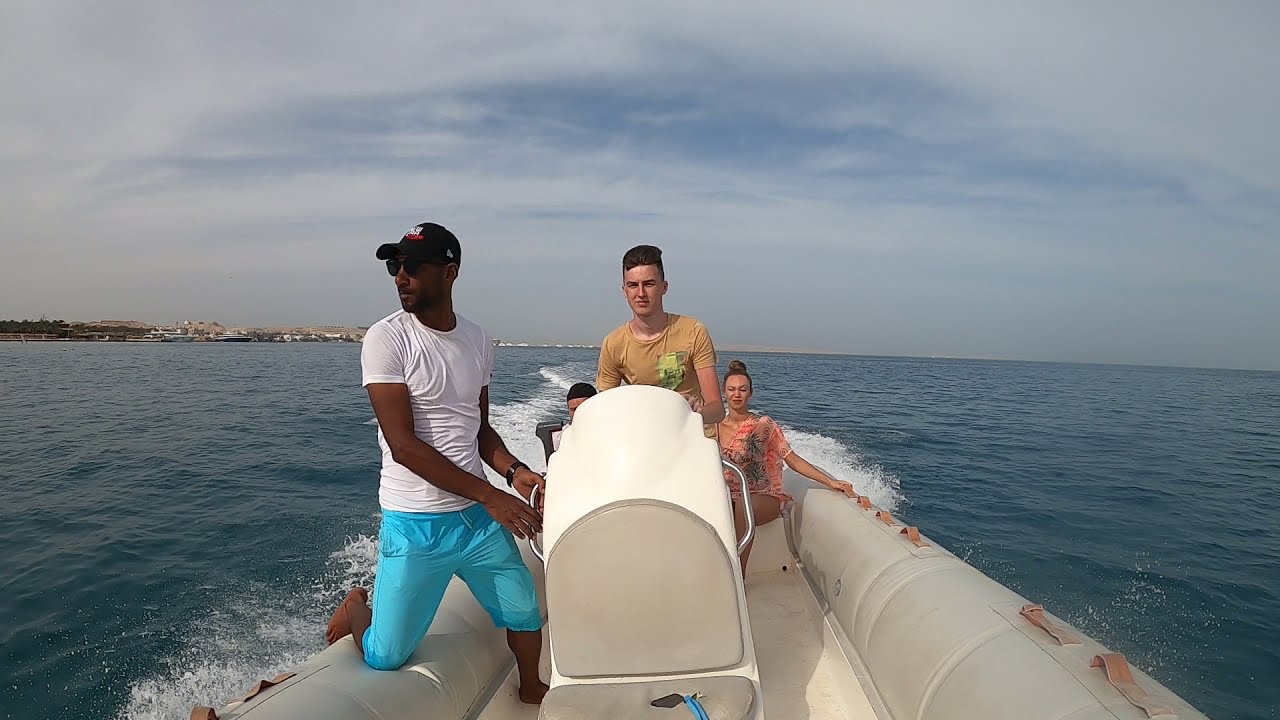The image depicts a group of people on a white speedboat navigating calm, blue ocean waters. The scene is set against a cloudy, overcast sky with wispy white clouds. In the background, there is a distant island with some buildings visible. At the center of the boat, a white man stands, possibly steering, dressed in a tan shirt. To his left, a black man is kneeling, wearing a black cap, white t-shirt, blue shorts, and sunglasses, gazing towards the water. Behind them, a white woman with blonde hair tied in a ponytail sits, holding the side of the boat. Another person, possibly a child, is partially visible next to her. The speedboat features a white compartment with silver handles near its center, possibly housing the engine, which the standing man seems to be holding onto.